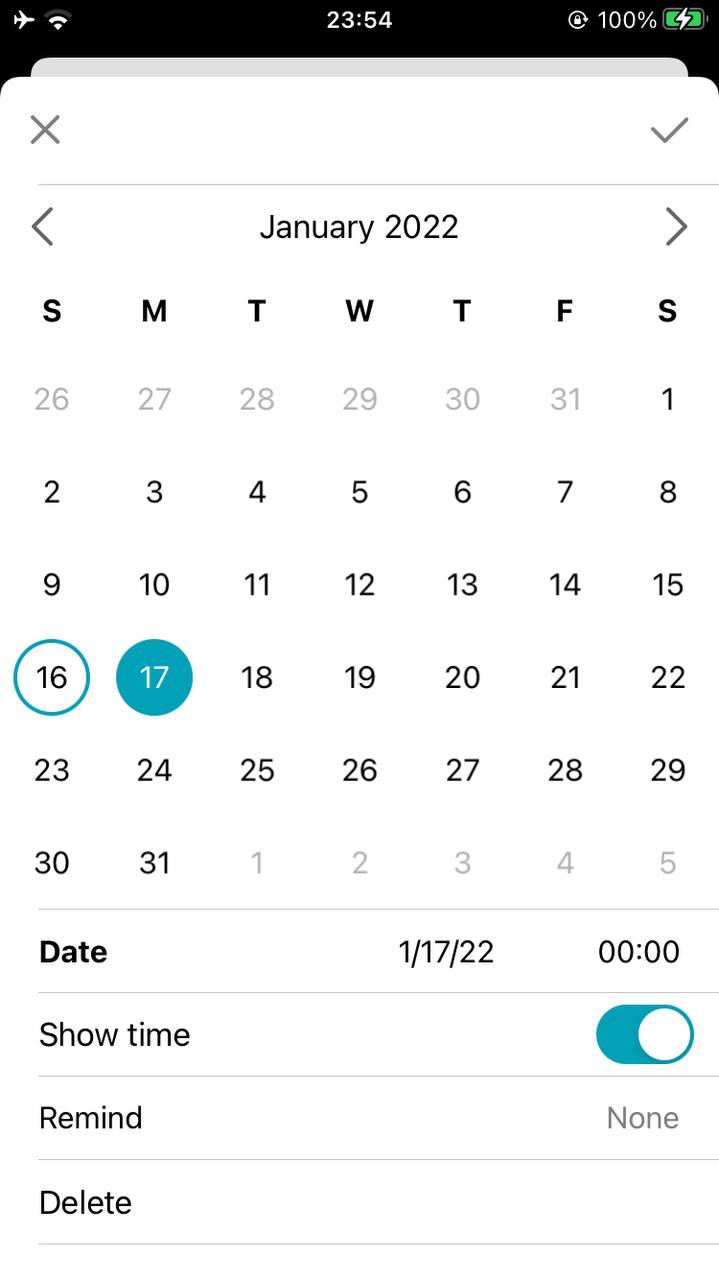In this detailed image, a calendar is prominently featured at the very top, overlaying a black rectangle and a smaller gray rectangle beneath it. The calendar itself has a white background. On the top left corner of the calendar, there is a black X, while the top right corner has a black checkmark. 

Along the top section of the calendar, there are arrows pointing left and right, flanking the text "January 2022." Below this header, the days of the week - labeled S, M, T, W, T, F, S - are spread out in bold letters across the calendar.

Each day of the week is accompanied by a column of dates:

- Under the first S: 26, 2, 9, 16, 23, 30.
- Under M: 27, 3, 10, 17, 24, 31.
- Under T: 28, 4, 11, 18, 25.
- Under W: 29, 5, 12, 19, 26.
- Under T: 30, 6, 13, 20, 27.
- Under F: 31, 7, 14, 21, 28.
- Under the second S: 1, 8, 15, 22, 29.

On the left side of the calendar, several labels are listed vertically: "Date," "Show Time," "Remind," and "Delete." Adjacent to the "Date" label, there is a specific date mentioned: "1/17/22."

Directly beside these labels, in the middle section, is a column that continues horizontally. There, the time "00:00" is displayed next to the "Show Time" label, with a blue dot indicating that the show time feature is active. Further to the right, next to the "Remind" label, is the word "None," denoting that there are no reminders set.